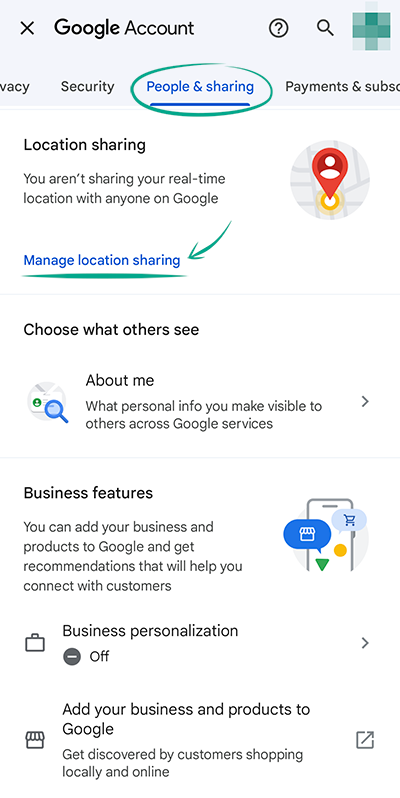**Caption:** 

The image is a screenshot from a mobile phone displaying a Google account page. At the top, the header includes the text "Google Account," an "X" button to the left, a question mark icon for help, a magnifying glass icon for search, and a blurred-out profile icon. Below the header are tabs labeled "Privacy," "Security," "People & Sharing," and "Payments & Subscriptions," with the "People & Sharing" tab circled in green, indicating it is currently selected.

The "People & Sharing" tab features several sections:
1. **Location Sharing**:
   - A blue link that says "Manage Location Sharing," underlined in green and marked with a green arrow.
 
2. **Choose What Others See**:
   - An "About Me" section explaining what personal information can be made visible to others across Google services, with a right-pointing arrow next to it.
 
3. **Business Features**:
   - An option to "Add your business and products to Google and get recommendations that will help you connect with others," marked with a briefcase icon. This section notes that business personalization is currently off and includes a right-pointing arrow.
   - Another option to "Add your business and products to Google," emphasizing that it helps get discovered by customers both locally and online, highlighted by a small shop icon.

Overall, the image provides a detailed overview of the "People & Sharing" settings within a Google account, with clear indications of where users can manage location sharing, visibility of personal information, and business-related features.